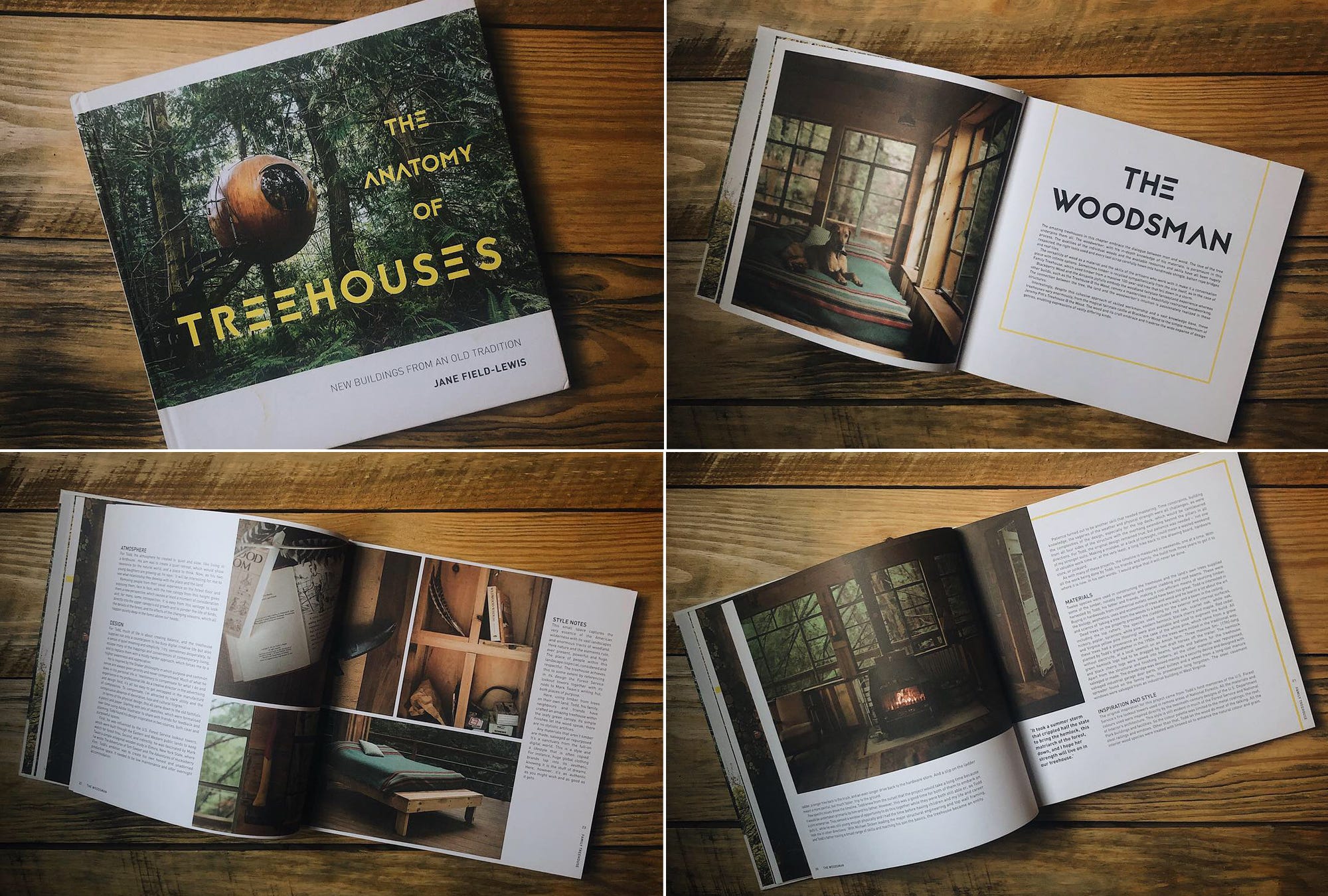A collage of four images is presented in a two-by-two grid. Each image features a book titled "The Anatomy of Tree Houses." The top-left image displays the front cover of the book. The top-right image shows the book open to a chapter titled "The Woodsman," accompanied by an illustrative photograph. The bottom-left image also has the book open, although the specific content of the page is not visible in detail. The bottom-right image again shows the book open, continuing to reveal its detailed illustrations and rich content related to tree houses.